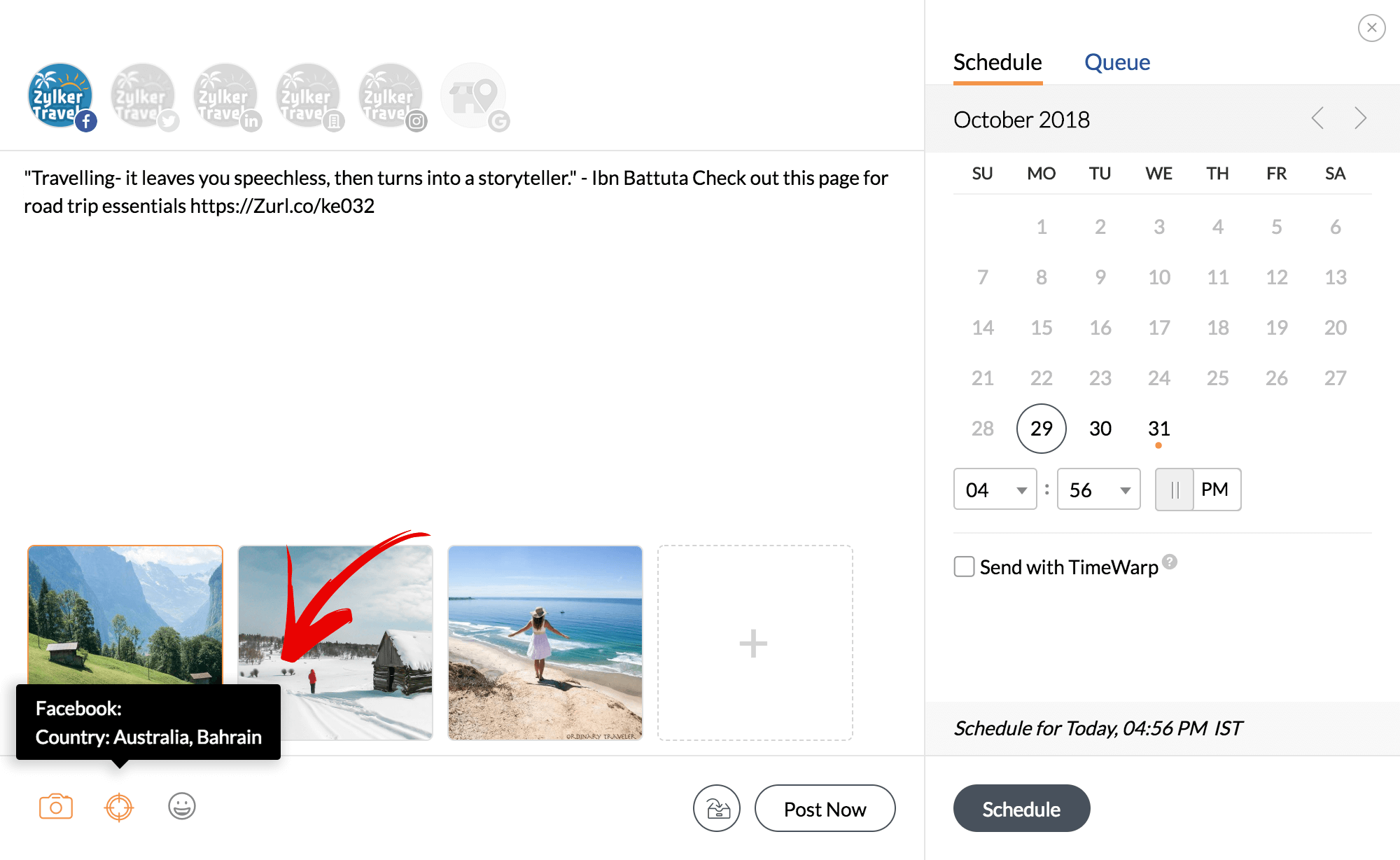A captivating screenshot of a travel-themed page on Facebook, adorned with an inspiring quote: "Traveling—it leaves you speechless, then turns you into a storyteller." The call to action encourages viewers to explore the page for road trip results and essential information. The interface reveals the platform as Facebook, with user settings indicating locations such as Australia and Bahrain. The post is meticulously scheduled for October 29th, 2018, at 4:56 PM, with options to send immediately or at a later time. Featured prominently in the post are three evocative images: the first captures an individual enjoying the serene ambiance of a beach, the second showcases a breathtaking snowy landscape, and the third reveals a lush, grassy plain set against the majestic backdrop of towering mountains. Each photograph contributes to a tapestry of diverse travel experiences, beckoning viewers to embark on their own adventures.